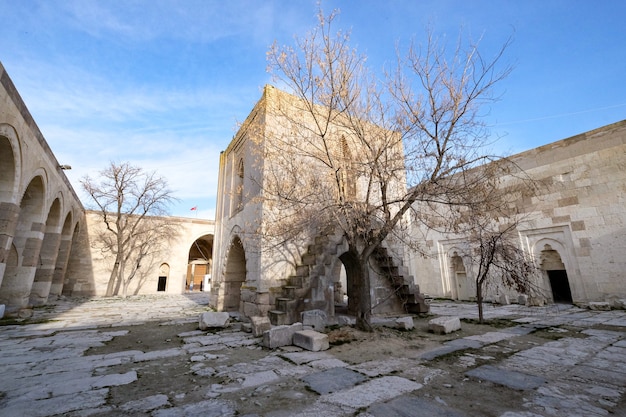The image depicts a dilapidated courtyard of an older building constructed from stone or brick. Central to the scene is a small, square brick structure featuring arched openings and staircases leading to a second level. The ground beneath and around this structure is composed of a stone paver surface, from which many stones have been removed or displaced, revealing dirt and rubble. On either side of the small structure, concrete stairs ascend, flanked by a tree that seems weathered and unhealthy, with sparse leaves. Multiple bare trees are scattered throughout the courtyard, suggesting a cold or wintery environment, though the sky above is a clear blue. Surrounding the courtyard are additional buildings, all with a similar stone appearance, some of which feature columns and decorative doors. Arched passageways can be seen on the left side and in the background, contributing to an overall sense of abandonment and decay that permeates the area.